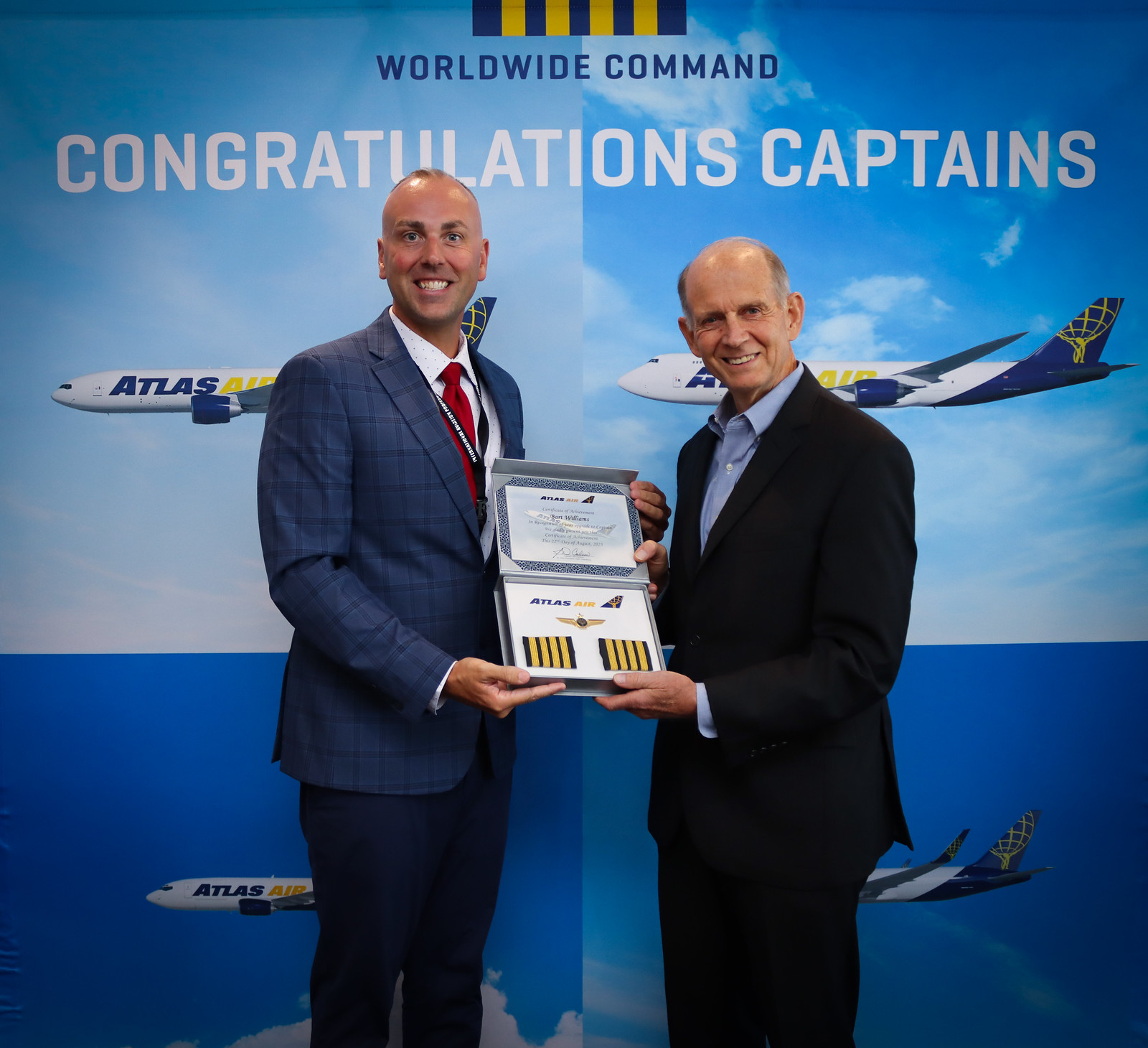This photograph features two men, dressed in professional attire—one in a blue suit paired with a red tie, and the other in a black suit—both standing prominently at the center of the image. They are holding certificates awarded by Atlas Air, commemorating their promotion to airline captains. The certificates, detailed with "Certificate of Achievement" and specifically mentioning Bart Williams, were awarded on August 22, 2023. Behind them, the backdrop showcases images of Atlas Air planes against a primarily blue background, adorned with white and blue text that reads, "Worldwide Command, congratulations captains." The background, combined with the attire of the men and their newly minted captain's bars—which display four yellow stripes on the blue background—emphasizes the celebratory nature of this award ceremony. The photograph captures the essence of the ceremony, highlighting the significant achievement of the men as they ascend to the prestigious rank of captains within Atlas Air.